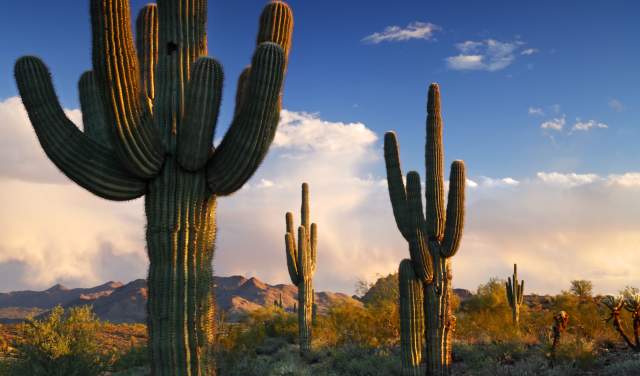In this striking desert landscape, towering cacti in shades of dark green and brown punctuate the terrain, their impressive heights commanding attention. Scattered among the arid ground, patches of greenery including grass and bushes add contrast to the scene. The backdrop features a rocky mountain range on the left, with smaller rocky hills extending to the right. The sky above transitions from a deep blue to a dense blanket of white clouds that dominate the middle of the image, creating a dramatic juxtaposition to the sparse desert below. The clouds, thick and fluffy, appear to hang like a blanket, adding depth to this visually captivating image.